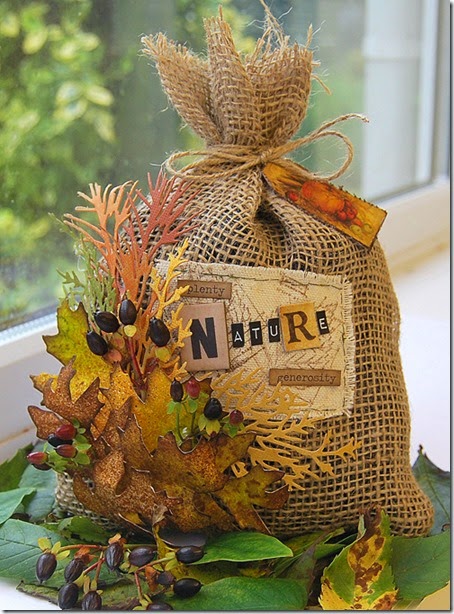The image depicts a decorative fall-themed burlap sack, intricately tied with twine and featuring a patch that spells out "Nature" with decorative, oversized letters on separate patches, as well as the words "Plenty" and "Generosity." This craft piece is adorned with artificial green leaves and yellow-brown leaves pasted to its sides, creating the impression of it resting naturally in an autumnal setting. Complementing the leaves are faux berries and seed branches positioned in front of the sack, enhancing the seasonal theme. The sack is centrally positioned on a windowsill inside someone's home, with daylight illuminating the scene, making it clear that this piece serves as a festive autumn decoration, likely sourced from a home goods store like Hobby Lobby, Target, or Home Depot.